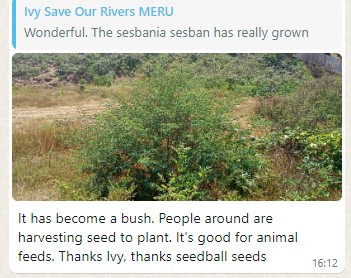The image is a screenshot from a mobile device showcasing an outdoor scene, likely from an online feed or comment. In the center of the image, there is a green bush surrounded by greenery, possibly located in mountains or a park. Behind the bush is a dirt road. The text on the screen is laid out with phrases both at the top and bottom of the image. At the top, it reads: "Ivy save our rivers Meru wonderful the sesbania sesban has really grown." Below the image, it continues: "It has become a bush, people around are harvesting seed to plant. It's good for animal feeds. Thanks Ivy, thanks seed ball seeds." The text uses various colors, including light blue for the phrase "Ivy save our rivers Meru" and black for the rest of the message. A timestamp at the bottom right corner indicates "16:12." The colors in the screenshot include white, gray, light blue, green, brown, and black, adding to the rich detail of the captured moment.